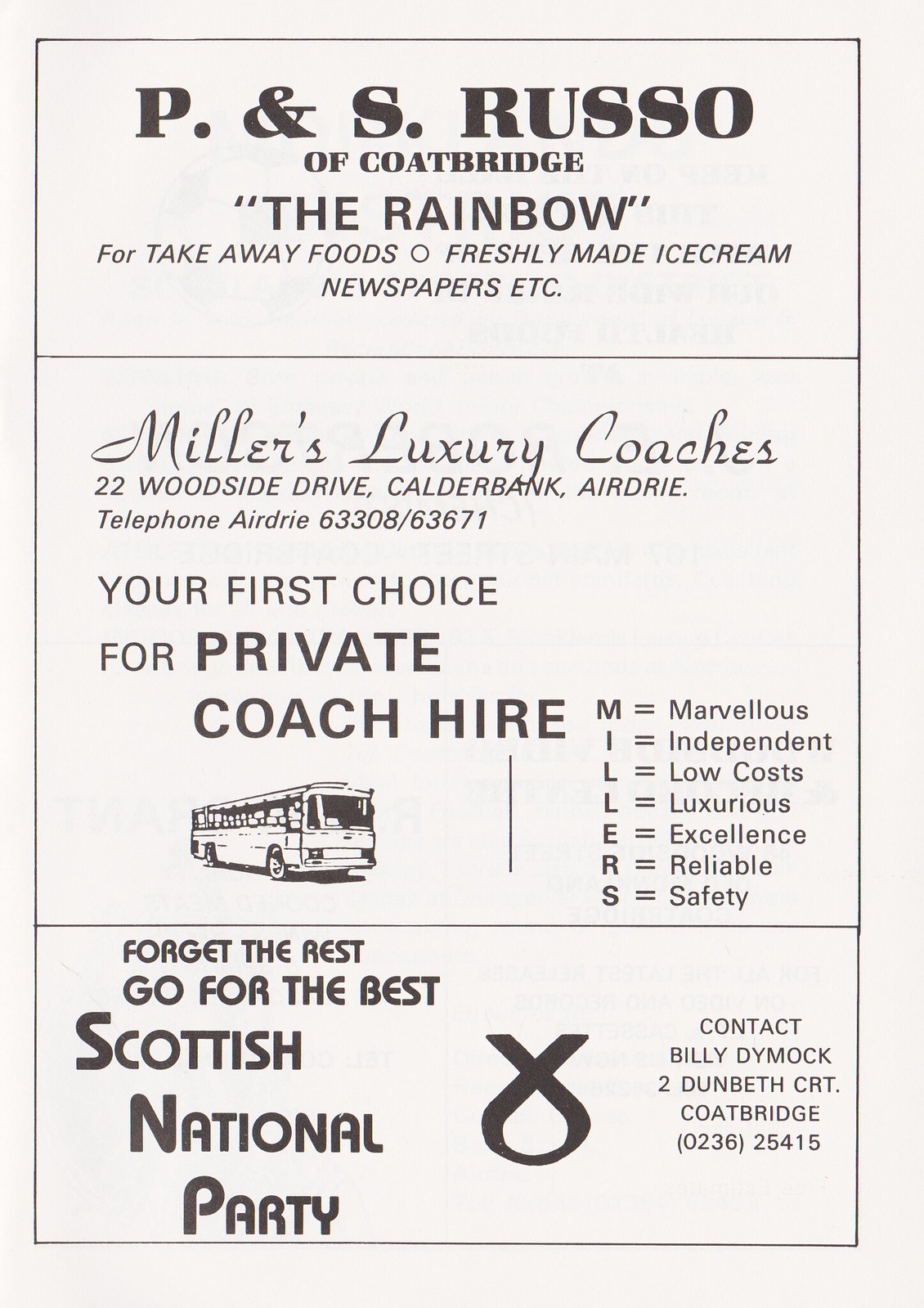The poster image, set against a light grey background with black text, is divided into three horizontal sections, each advertising distinct services. 

In the top section, the text reads "P&S Russo of Coatbridge," branded as "The Rainbow" for takeaway foods, featuring freshly made ice cream and newspapers. 

The middle section is dedicated to "Miller's Luxury Coaches," listing their address as 22 Woodside Drive, Calderbank, Airdrie, with the telephone number Airdrie 6330863671. Described as "Your first choice for private coach hire," this section emphasizes attributes like marvelous, independent, low-cost, luxurious, excellence, reliable, and safety. It also includes a drawing of a bus.

The bottom section promotes the "Scottish National Party" with the slogan, "Forget the rest, go for the best." Contact information here lists Billy Dymock at 2 Dunbeth Court, Coatbridge, with the phone number 0236-25415. The section also features a ribbon-like emblem.

Overall, the poster effectively advertises the services of a local business, a luxury coach service, and a political party, each with clear contact details and distinctive branding elements.